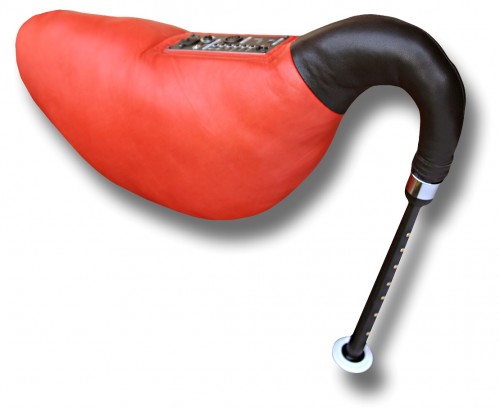The image shows a close-up of a unique, kidney-shaped device with a primarily red body and a distinctive black handle-like extension. The device appears to have a control panel on its red part, featuring buttons and knobs, indicating it may serve a mechanical or electronic function. The black handle extends downward into a long black tube, accented by a silver ring near the base. This tube has a series of six or seven holes along its length and terminates in a flat, white circular surface. The overall shape and design suggest possible uses ranging from a specialized tool, a musical instrument, or even a handheld vacuum. The device casts a shadow behind it, and it is set against a completely white background, allowing its details to stand out clearly.